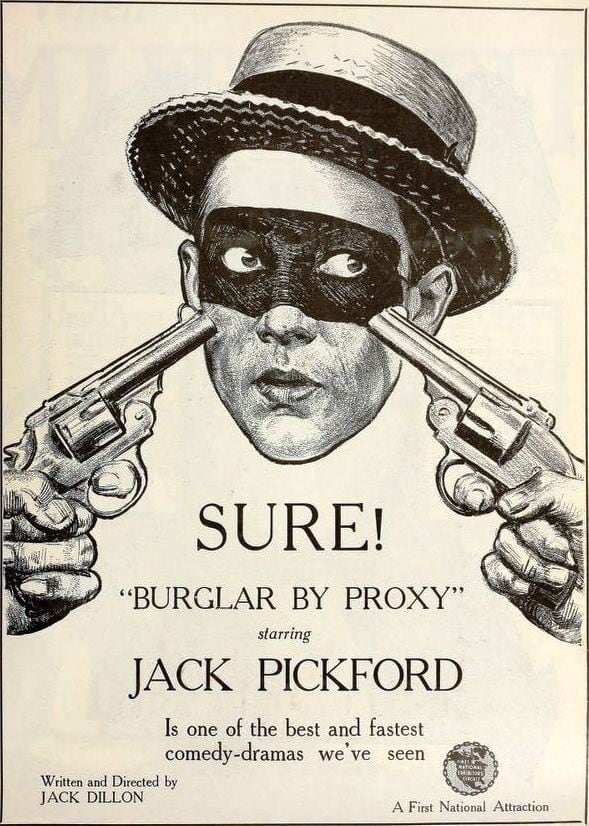The image is a detailed black-and-white sketch with text on a cream-colored background surrounded by a narrow black border, resembling a vintage movie poster or playbill. Dominating the top half of the composition is a meticulously drawn floating head of a man with fair complexion and brown hair. The man is adorned with a black eye mask that conceals his eyes and nose, similar to those worn by old-time burglars, with his wide-open eyes peering through. He wears a textured straw Panama hat featuring a black band at the base, underscoring the period feel of the illustration.

Standing out distinctly are two revolvers aimed directly at the man's face, adding a dramatic and tense element to the artwork. Beneath the portrait, bold text proclaims "SURE!" followed by "Burglar by Proxy" in quotations. The accompanying text credits Jack Pickford as the star and emphasizes the production's acclaim with the phrase "is one of the best and fastest comedy dramas we've seen." Further down, it notes that the piece was written and directed by Jack Dillon, and it identifies the production as "a First National Attraction."